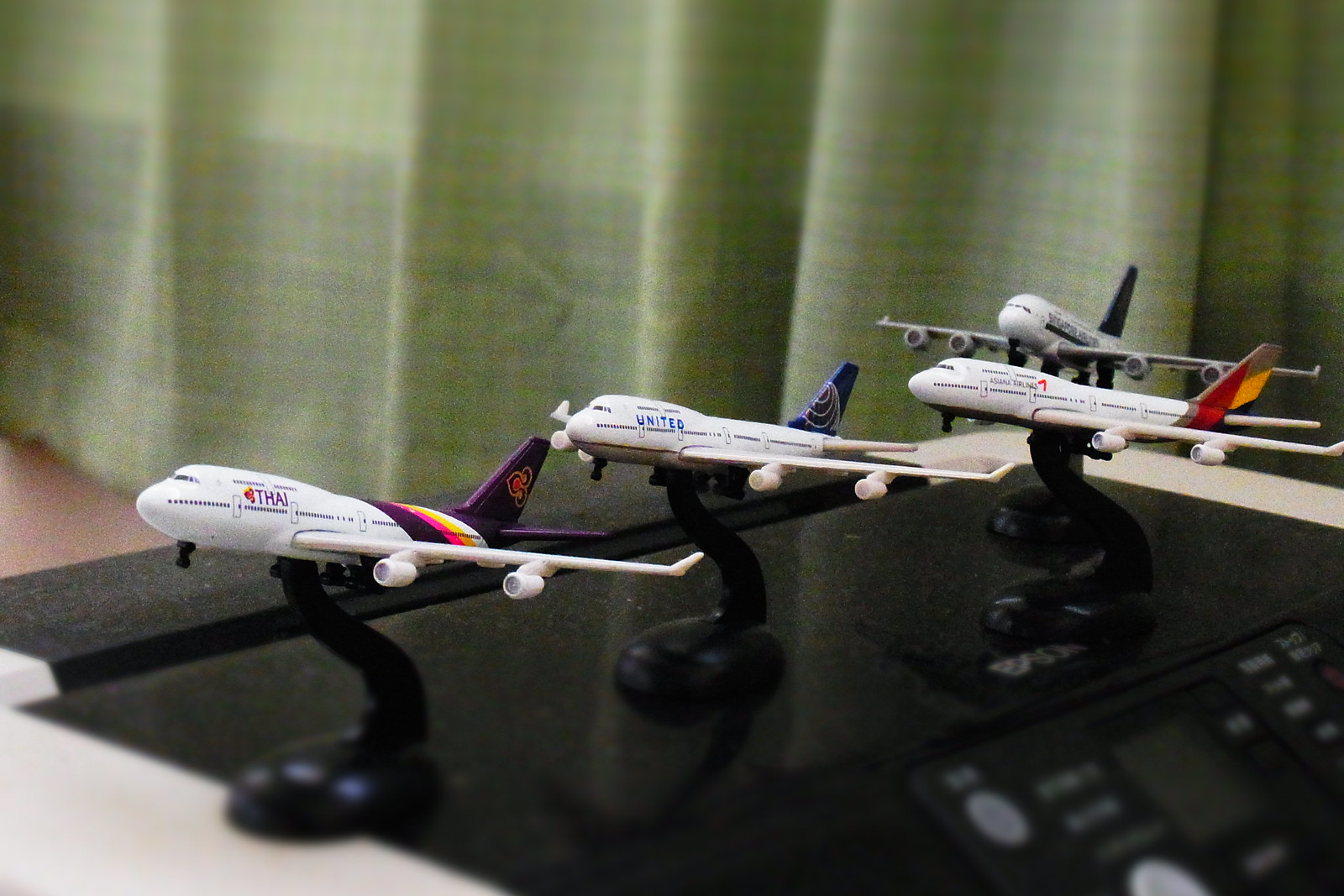This close-up photograph captures the top of a black printer, slightly out of focus in the bottom right corner where its digital screen and buttons are visible. On top of the printer sit four miniature airplanes, each mounted on a curved black plastic stand that mimics the planes in flight at a 45-degree angle. The nearest plane to the left is a white Thai Airlines jet with a purple tail accented by red and yellow stripes. Next is a white United Airlines plane with a distinctive blue tail featuring a globe design. The third plane, also white, has an intricate tail pattern of red, brown, and yellow, although its airline name is unreadable. The farthest plane is white with a dark-gray tail. The background of the image is dominated by a green plaid curtain that spans from the left to the right-hand side, and hints of what might be bed material in shades of green are visible, suggesting the image was taken indoors, possibly in a bedroom.